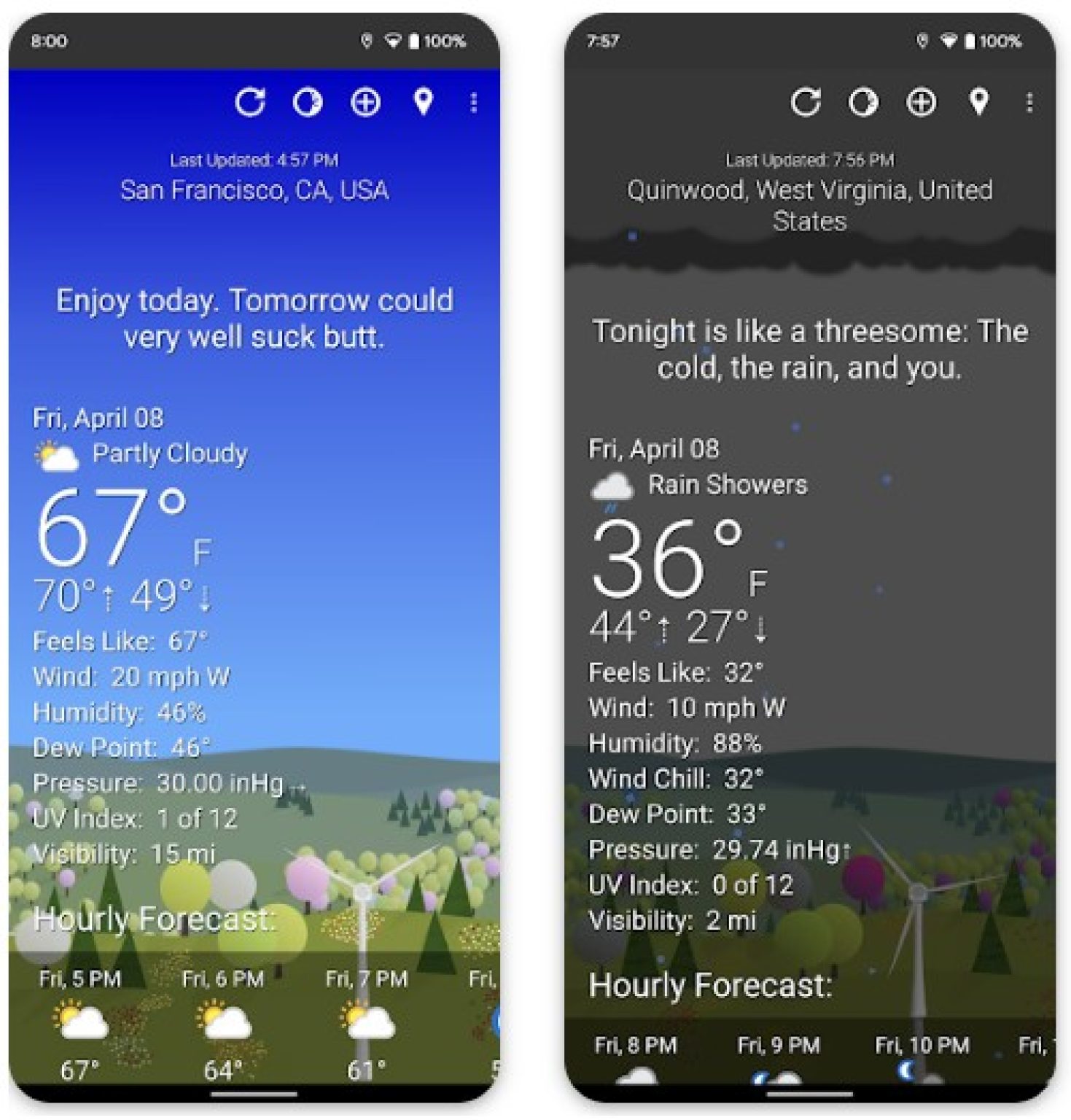The image consists of two side-by-side phone screenshots displaying detailed weather information for different locations.

**Left-Hand Side:**
- **Background:** Blue and sunny.
- **Temperature:** 67 degrees Fahrenheit.
- **Additional Info:** High, low, "feels like" temperature, wind speed and direction, humidity, dew point, pressure, UV index, and visibility.
- **Hourly Forecast:** Displayed at the bottom.
- **Top of Screen:** Includes the time (left-hand side), maps indicator, Wi-Fi indicator, and battery indicator.
- **Location:** San Francisco, California, USA, in white text centered at the top.

**Right-Hand Side:**
- **Background:** Rainy and darker, indicating nighttime.
- **Center Text:** "Tonight is like a threesome, the cold, the rain, and you."
- **Date and Weather:** Friday, April 8th, rainy showers, 36 degrees Fahrenheit.
- **Additional Info:** High, low, "feels like" temperature, wind speed and direction, humidity, wind chill, dew point, pressure, UV index, and visibility.
- **Hourly Forecast:** Displayed at the bottom.
- **Top of Screen:** Includes the time, maps indicator, Wi-Fi indicator, and battery indicator.
- **Update Time and Location:** Last updated at 7:56 PM, Quinnwood, West Virginia, USA, in white text centered at the top.

Both screenshots have white text, with a white border separating the images. The left side shows a sunny, daytime scene, while the right side depicts a darker, rainy night.